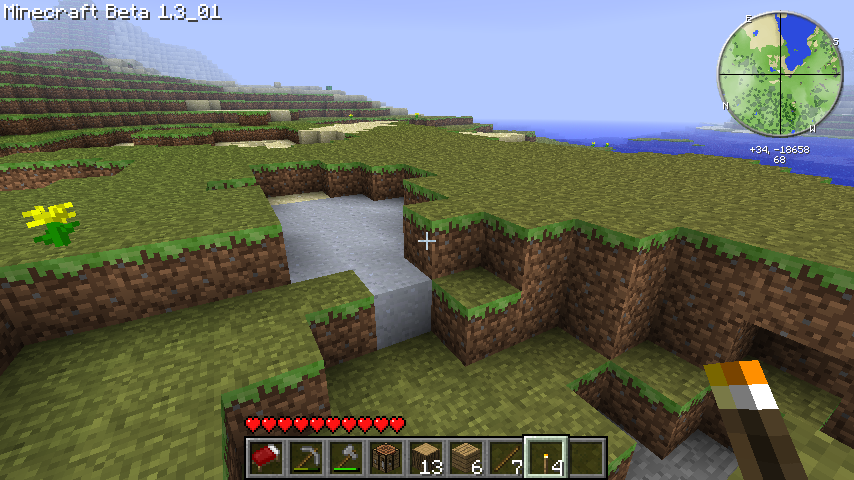A detailed screenshot of an early Minecraft Beta 1.3-01 version. In the upper left corner, the version is clearly indicated. The bottom of the screenshot showcases various avatar-related buttons and a series of earned hearts symbolizing health status. The upper right corner features a small photo resembling a telescopic sight, focusing on a specific area within the image. The central part of the screenshot displays a fortress-like structure, consisting of brick or paver walls, and numerous climbable areas that lead to horizontal gray surfaces and additional ascent points. In the background, multiple terraces ascend upwards, ultimately reaching a mountainside adorned with more terraces. The upper right center of the image reveals a distant view featuring water and a horizon set against a light blue overcast sky. This captures the essence of a very early Minecraft experience during its Beta 1.3 phase.